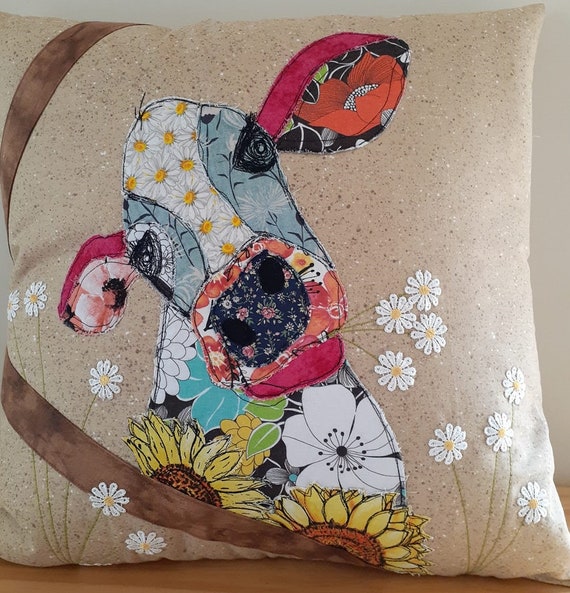This detailed indoor photograph captures a beige pillow with a slightly grainy texture against a white wall. The pillow features an intricate, quilt-like design of a cow, seemingly pieced together from various cloths. The cow's eyes are surrounded by a bluish-gray fabric, with its snout made from black cloth adorned with floral prints. Pinkish fabrics highlight its ears and the lower part of its mouth. The cow is depicted holding white daisies in its mouth, with more daisies stitched around the sides of the pillow. In the background, sunflowers and other colorful flowers, including lilies, are intricately sewn into the fabric. A distinctive brown band starts from the bottom middle of the image, curving gracefully to the top left corner. There is no text present on the image.